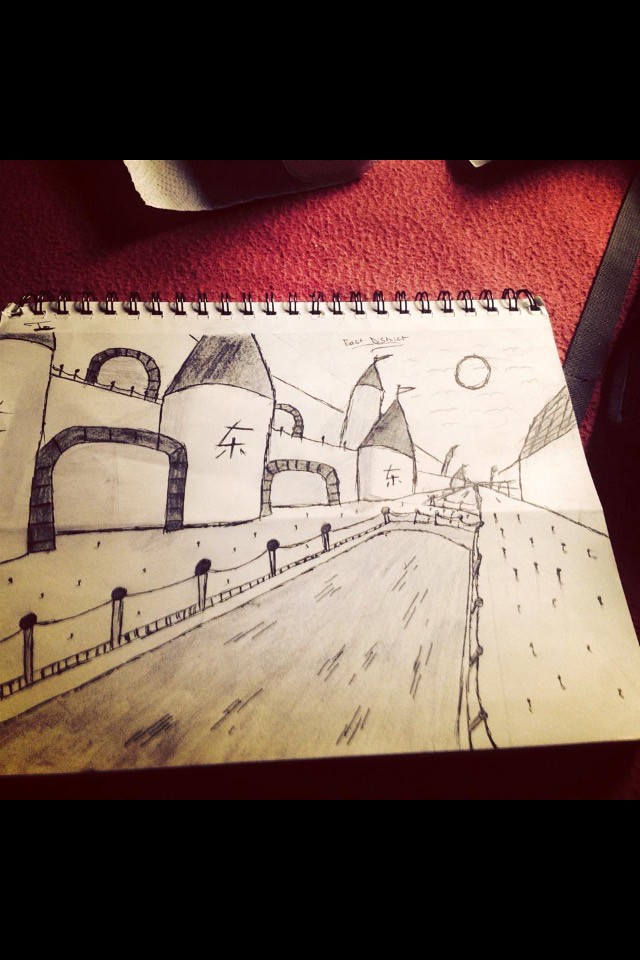The image captures a photograph of an open sketch notebook laid across a red, textured surface that resembles felt or a bumpy fabric. The sketch itself, rendered entirely in black and white pen, depicts a medieval-themed scene dominated by a river running through the middle. On either side of this waterway, there are intricate buildings, likely representing a castle and adjacent structures. The castle stands on the left with detailed arches, roofed towers adorned with flags, and several doorways and windows. Protective fencing and walkways border the river, and small dots representing people are scattered along these paths. There is notably Asian writing on some of the buildings, adding an exotic flair to the medieval vista. In the distant background, a sun or moon is visible in the sky, accompanied by a few birds. The artist's signature is also discernible at the top of the sketch, though it is somewhat illegible. The overall scene is rich in detail, creating a vivid portrayal of a bustling, fortified settlement.